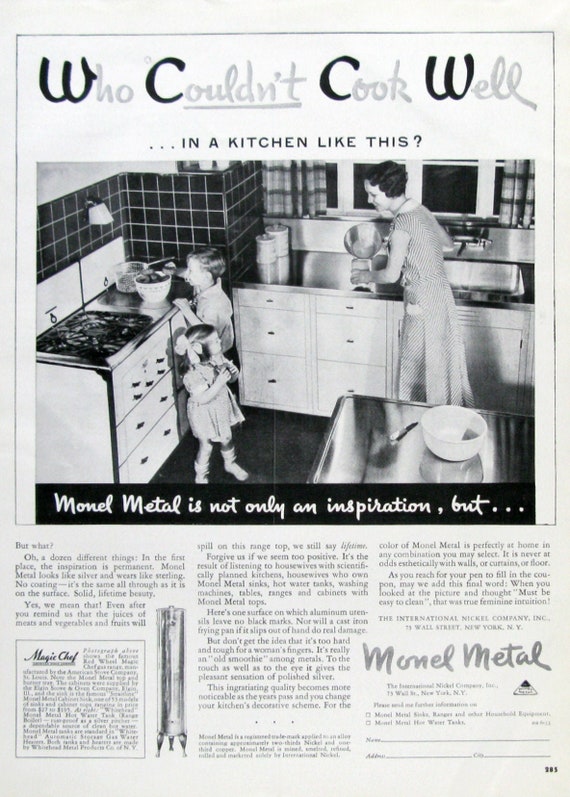This black and white advertisement, seemingly from the 1940s or 1950s, presents a nostalgic yet innovative kitchen scene under the headline, "Who Couldn't Cook Well In a Kitchen Like This." Central to the ad is a detailed photograph of a mother preparing food, with her two children eagerly observing and engaging in the kitchen activities. The kitchen, equipped with a sink, countertops, and a stove, evokes a sense of vintage charm and functionality. The mother is depicted holding a bowl, attracting the curious gaze of a boy peering into it, while a girl stands nearby. The ad celebrates Monel Metal, described as "not only an inspiration," with the bottom section featuring approximately twelve informative paragraphs extolling its benefits and modern appeal, making it a quintessential feature of what would have been considered a "space-age" kitchen at the time.